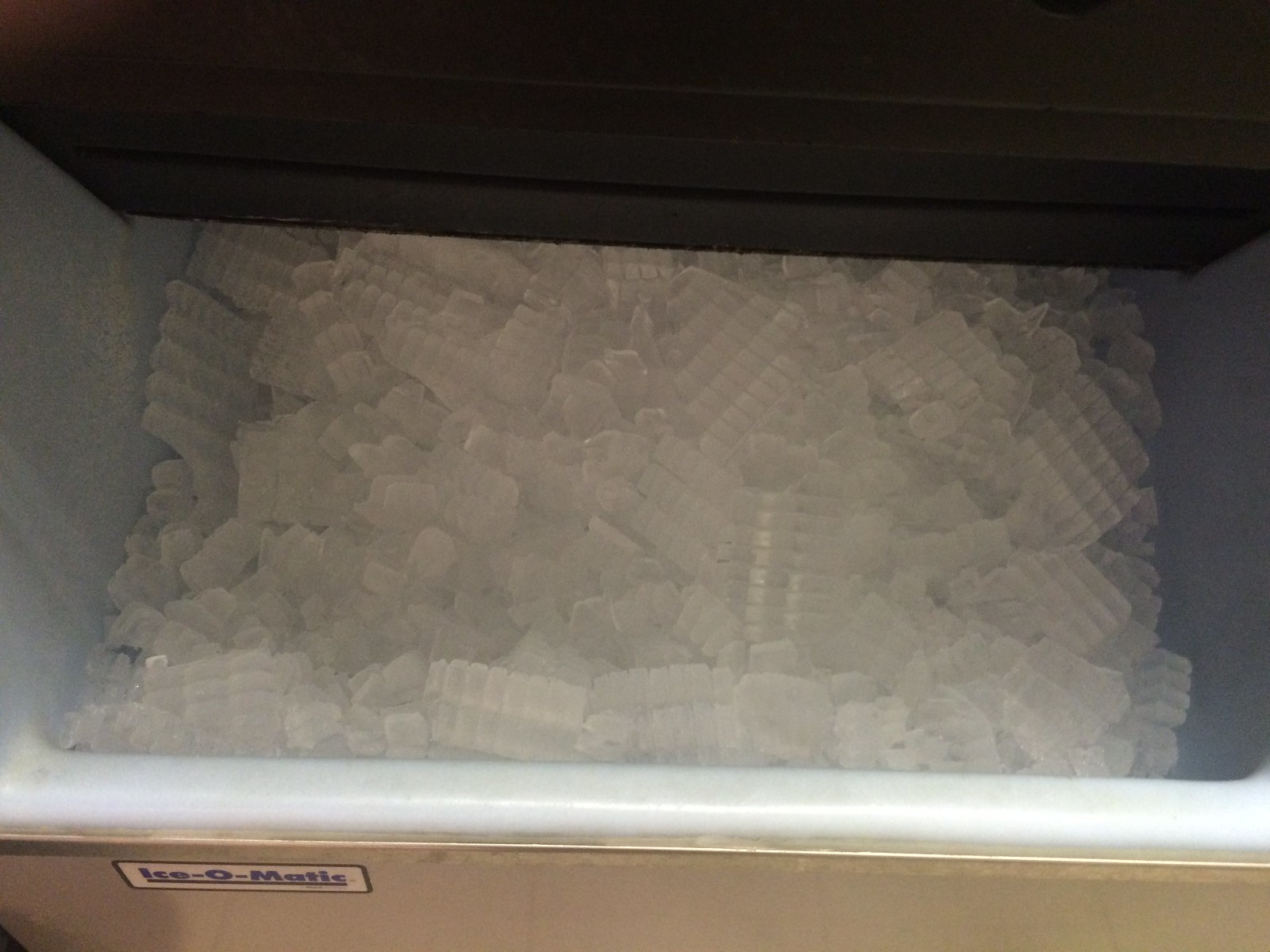The photograph captures the inside of an Ice-O-Matic ice chest, with a black lid flipped open. The ice chest is notably vintage in style with a stainless steel front, white trim, and tan walls. The interior reveals ice cubes, some of which are clear and slightly fogged, broken up yet stuck together in rows, as if freshly extracted from an ice tray. This commercial-grade ice machine, which appears to be less than half full, creates a sense of readiness to chill drinks or other items. The bottom left corner of the image prominently displays the blue Ice-O-Matic logo. The overall setting suggests the photo was taken indoors, perhaps in a restaurant or similar establishment, with a black wall or cabinet edge visible above the chest.